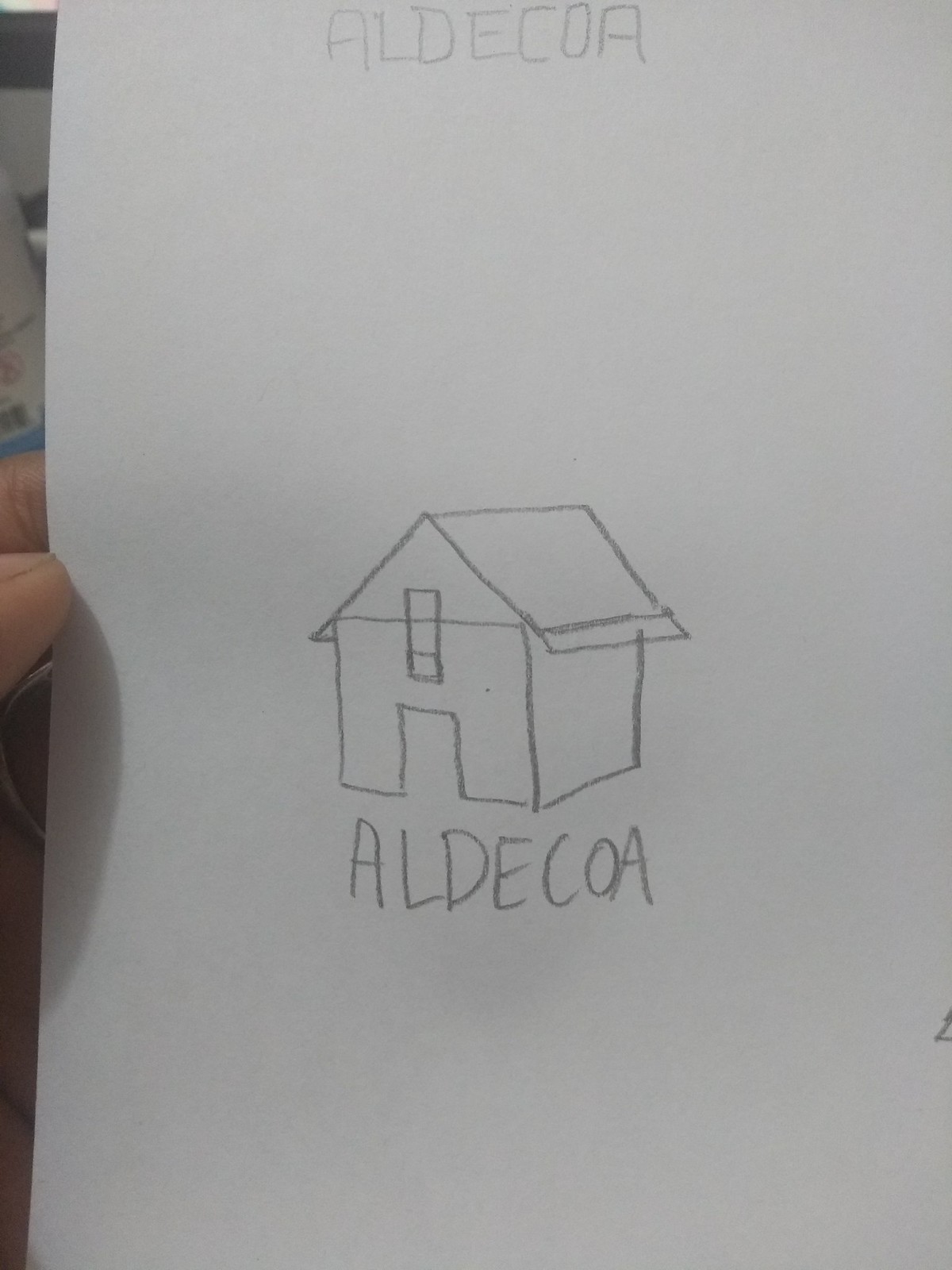A piece of white paper nearly fills the entire frame of the image. Positioned at the center left edge, a person's thumb gently touches the paper. At the top of the paper, the word "ALDECOA" is written in capital letters using a pencil. In the middle of the paper, there is a simple pencil drawing of a house, resembling a basic stick-figure representation. The house includes an open doorway, a single window above, and a roof, and it is slightly rotated towards the bottom left of the image, giving it a 3D perspective. Below the house, the word "ALDECOA" is repeated in the same pencil writing.